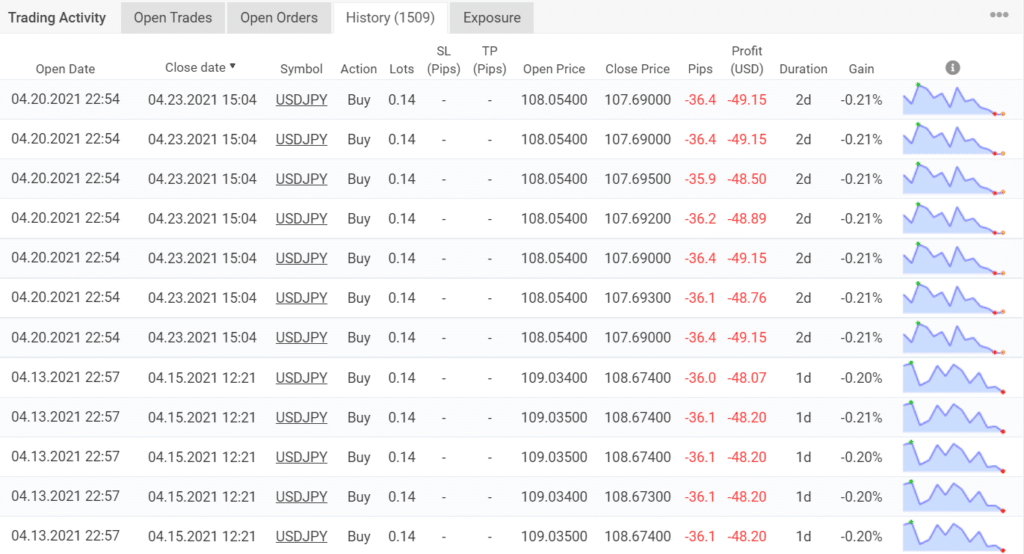This image showcases a trading activity page with multiple tabs at the top, including "Trading Activity," "Open Trades," "Open Orders," "History" (the current tab), and "Exposure." The interface is highly detailed and organized in a vertical list format, featuring multiple columns with the following headers: "Open Date," "Close Date" with a drop-down arrow, "Symbol," "Action," "Lots," "SLPIPS," "TPPIPS," "Open Price," "Close Price," "PIPS," "Profit," "U.S. Dollar," "Duration," and "Gain." 

At the end of each row, there's a graph indicated by a blue line that visualizes the movement.

Specific details include:
- All entries except for one have the open date of 4/20/2021, with timestamps of 22:54 for the first seven entries.
- The following four entries have an open date of 4/13/2021 at 22:57.
- The uniformity continues with all symbols listed as USDJPY.
- The action indicated in all entries is "Buy," and the lot size is consistently 0.14.
- The data columns for each trade also show their respective open and close prices, PIPS, profit (in U.S. dollars), duration, and gain values.

This detailed occupational image captures the systematic layout and specific data points crucial for trading analysis.